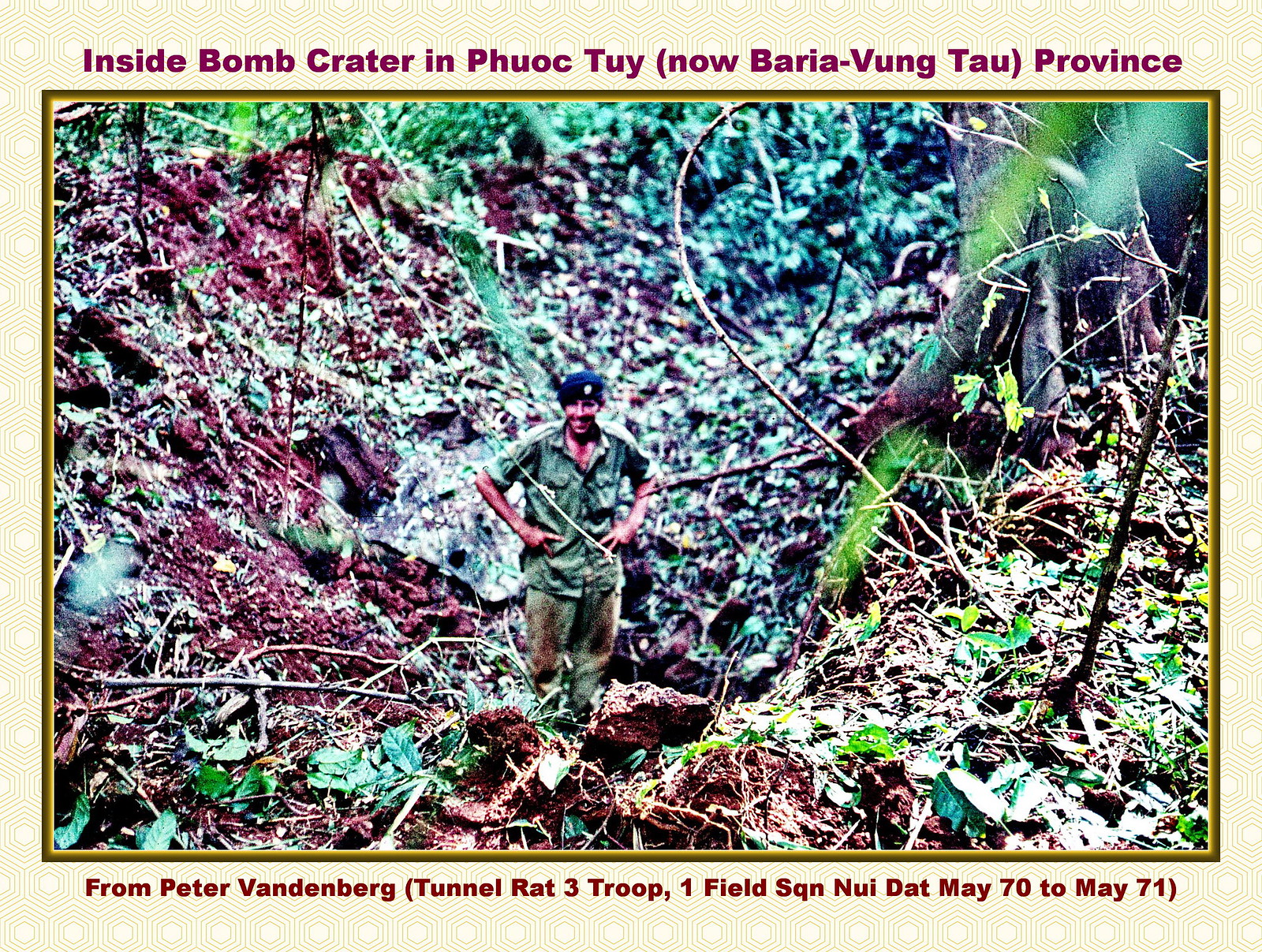The rectangular photograph features a scene labeled across the top in brown text: "Inside Bomb Crater in Phuoc Tuy (now Baria-Vung Tau Province)". The bottom text, in red, reads: "From Peter Vanderburg, Tunnel Rat 3, Troop 1, Field Squadron, Nui Dat, May 70 to May 71". The image, set against a light green border with yellow or tan circles and a subtle honeycomb pattern, shows a man with tanned skin standing at the center in a jungle environment. He is wearing a blue beret with a yellow pin, a green button-up shirt with the sleeves rolled above his shoulders, and dirty green trousers. With his hands on his hips, he’s smiling directly at the camera. Sunlight filters through the dense foliage, revealing a large tree trunk to his right and emphasizing the overgrown, leafy surroundings, which seem to be at the bottom of a depression or ditch.